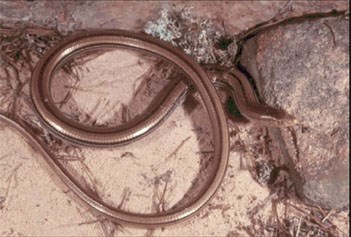This color photograph provides a detailed top-down view of a long, thin snake with a shiny, metallic bronze or silver-gray body that reflects the light. The snake features dark brown stripes running lengthwise from its head to its tail. In the image, the snake is partially curled into a loop with its head resting on a large stone, while its body extends across a sandy surface decorated with scattered twigs, pine needles, grass, and small rocks. The snake appears to be either hiding or preparing to move, captured in a moment of stillness amidst its natural, earthy surroundings.